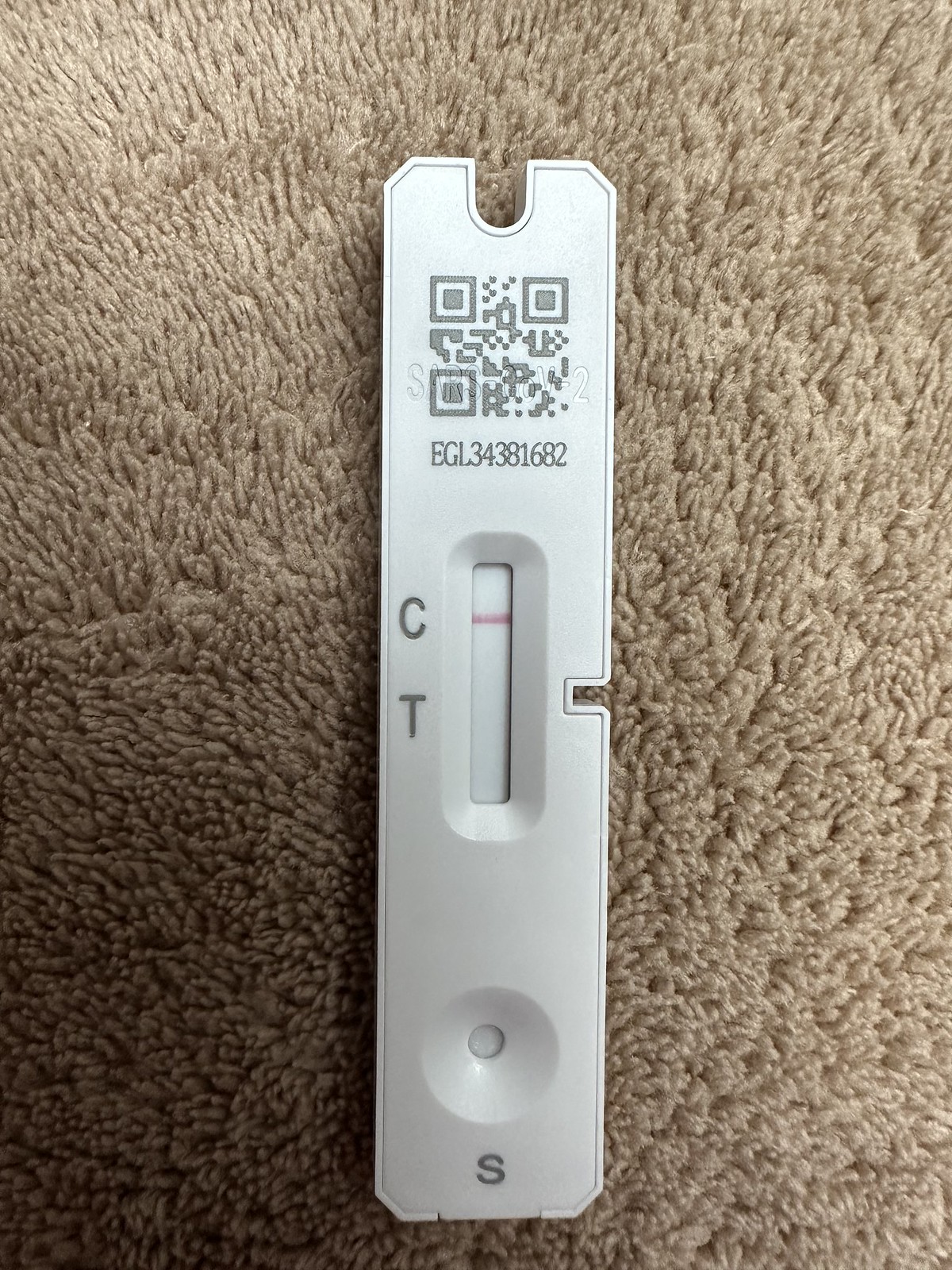A close-up image shows a white rapid COVID-19 test kit on a grayish-beige carpet background, oriented vertically. At the top of the rectangular plastic device, there is an engraved QR code with the text "SARS-COV-2" embedded above it, and alphanumeric code "EGL34381682" printed just below. Centrally located beneath the QR code, a small rectangular window displays the test results. To the left of this window, labels "C" and "T" run vertically beside it. A red line appears next to the "C," indicating a negative result, as there is no line next to the "T." At the bottom of the device, there is a small well marked with an "S" located centrally beneath it, signifying the sample deposition area. This detailed depiction underscores the functionality and result interpretation of the rapid test.